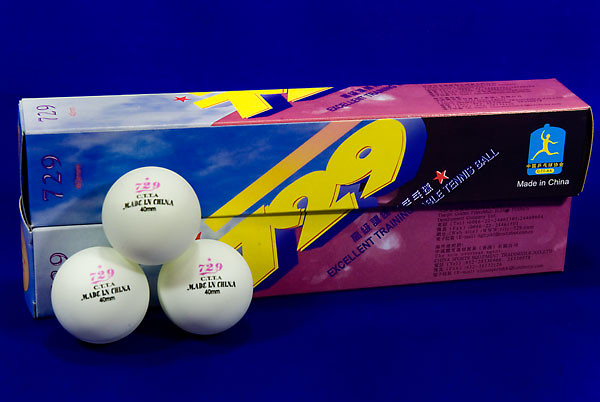This close-up product photo, set against a dark blue background with subtle black markings, showcases a pair of horizontally stacked rectangular boxes, each about a foot long, and features training ping pong balls. The boxes have a distinct blue sky design on the top left portion, transitioning to a black and pink color scheme on the side panels, and are adorned with yellow and pink logos displaying the number "729". Prominent black text and some Mandarin characters are also present, along with a "Made in China" label on the top right. In front of the boxes, a small pyramid of three white ping pong balls is arranged, with two at the bottom and one stacked on top. Each ball is marked with the same "729" in pink and additional black text, indicating they are made in China and measure 40 millimeters in size.